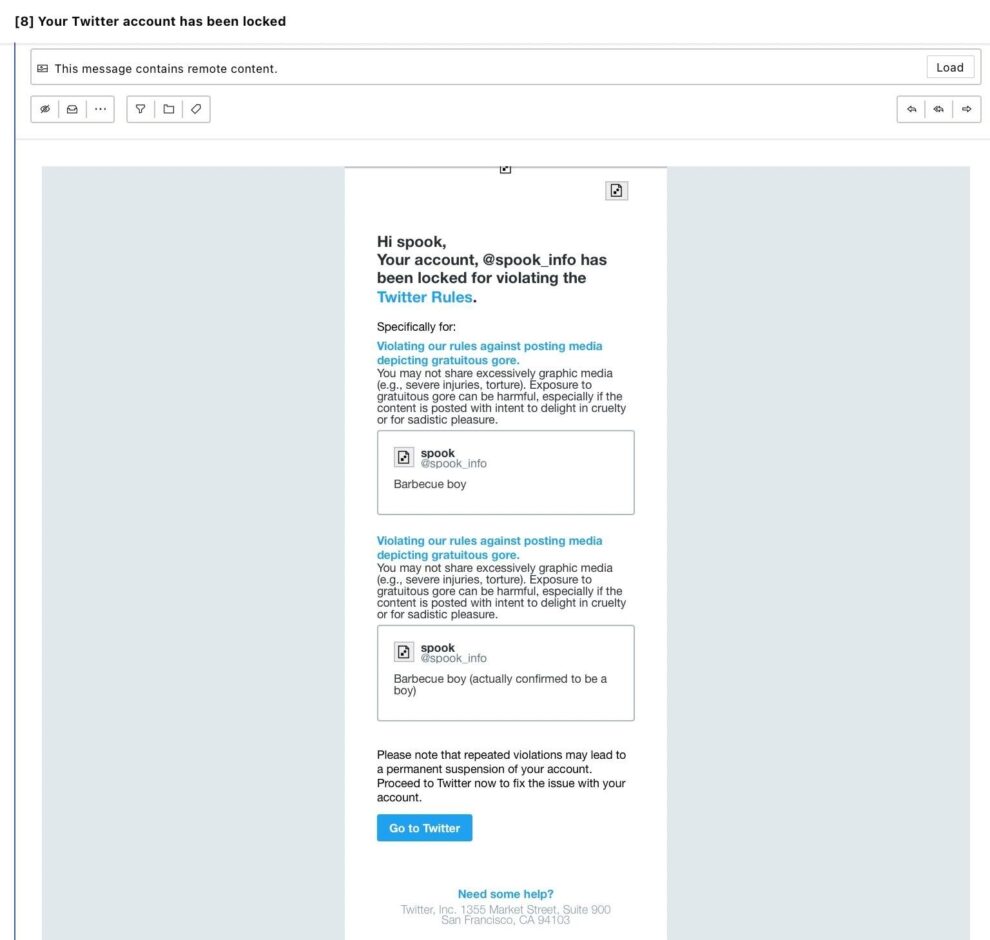This screenshot captures the notification of a locked Twitter account, detailing the following elements:

In the upper left-hand corner, there's a bolded number "8" in brackets. To the right, in bold, black text, reads "Your Twitter account has been locked." Below this heading are two thin, gray horizontal lines.

Next, there's a long, horizontal rectangle outlined in gray. On the left side, the text "This message contains remote content" appears in black. To the right is a "Load" button.

Beneath this are several small squares containing icons, including a file icon and an ellipsis, with three additional icons on the right side.

Following this, there's a large, light gray square with a centered vertical white rectangle. At the top left of this rectangle, in bolded black text, it says "Hi Spook," followed by "Your account @spook_info has been locked for violating the" with "Twitter Rules" in blue text. Specifically, the violation is labeled "Four."

Below this, there are two lines of blue text and five lines of black text explaining the violation. Another gray-outlined rectangle follows, containing the bolded black text "Spook" on top, and "Barbecue Boy" beneath it.

Lastly, there are two more lines of blue text, followed by additional black text listing the specific violations.